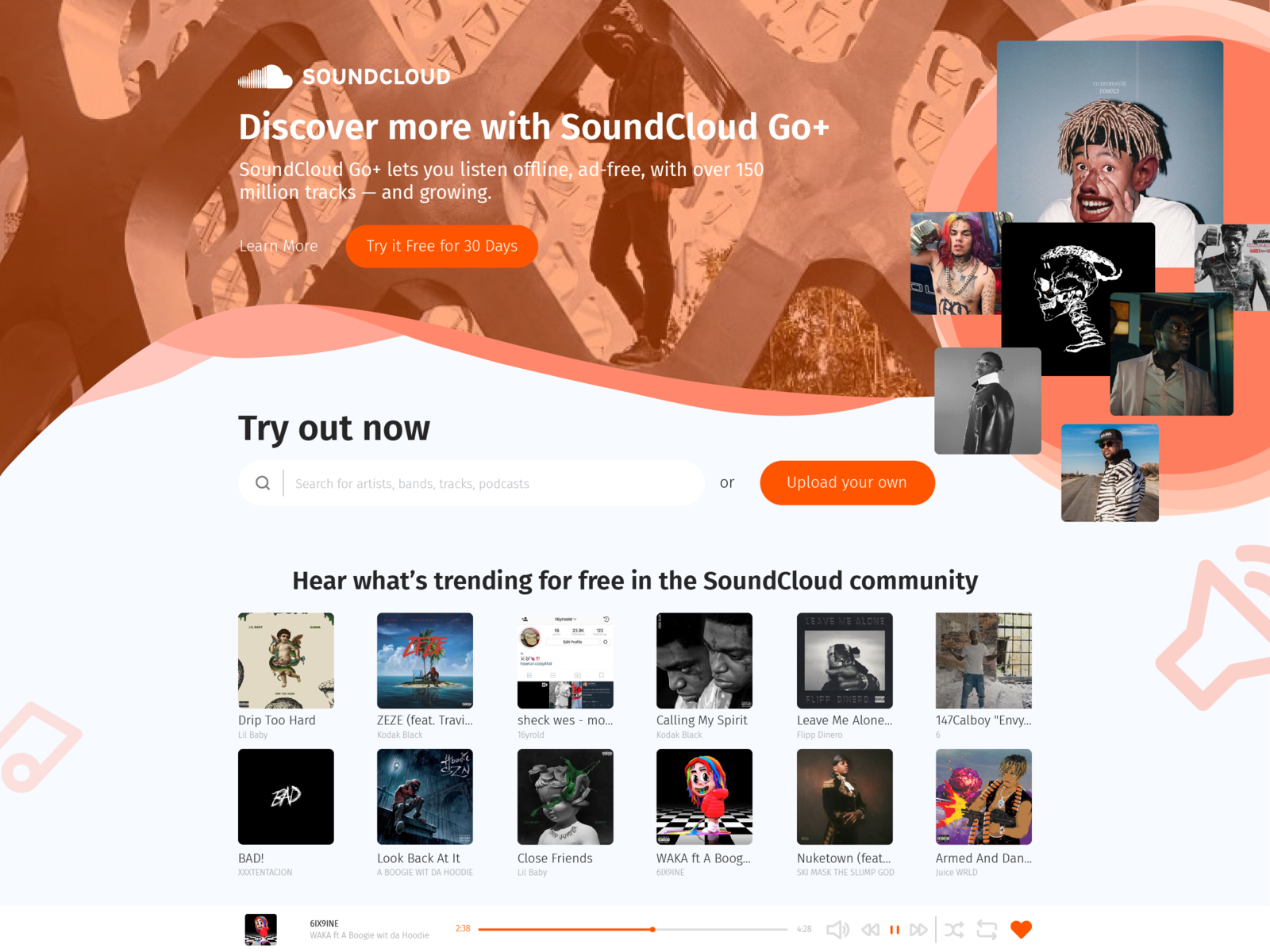The screenshot showcases the SoundCloud website interface. At the top, prominently, is the SoundCloud logo. Below the logo, a headline advertises SoundCloud Go+, which promises users the ability to listen offline and ad-free to an extensive library of over 150 million tracks, with more being added regularly. On the left side, there's a "Learn More" link, while on the right, a button invites users to "Try it free for 30 days." Positioned below this, another call-to-action button reads "Try out now." A search bar is also visible, encouraging users to "Search for artists, bands, tracks, podcasts." Adjacent to the search bar, the word "or" is displayed, leading to an orange box on the far right labeled "Upload your own," allowing users to upload their own audio content.